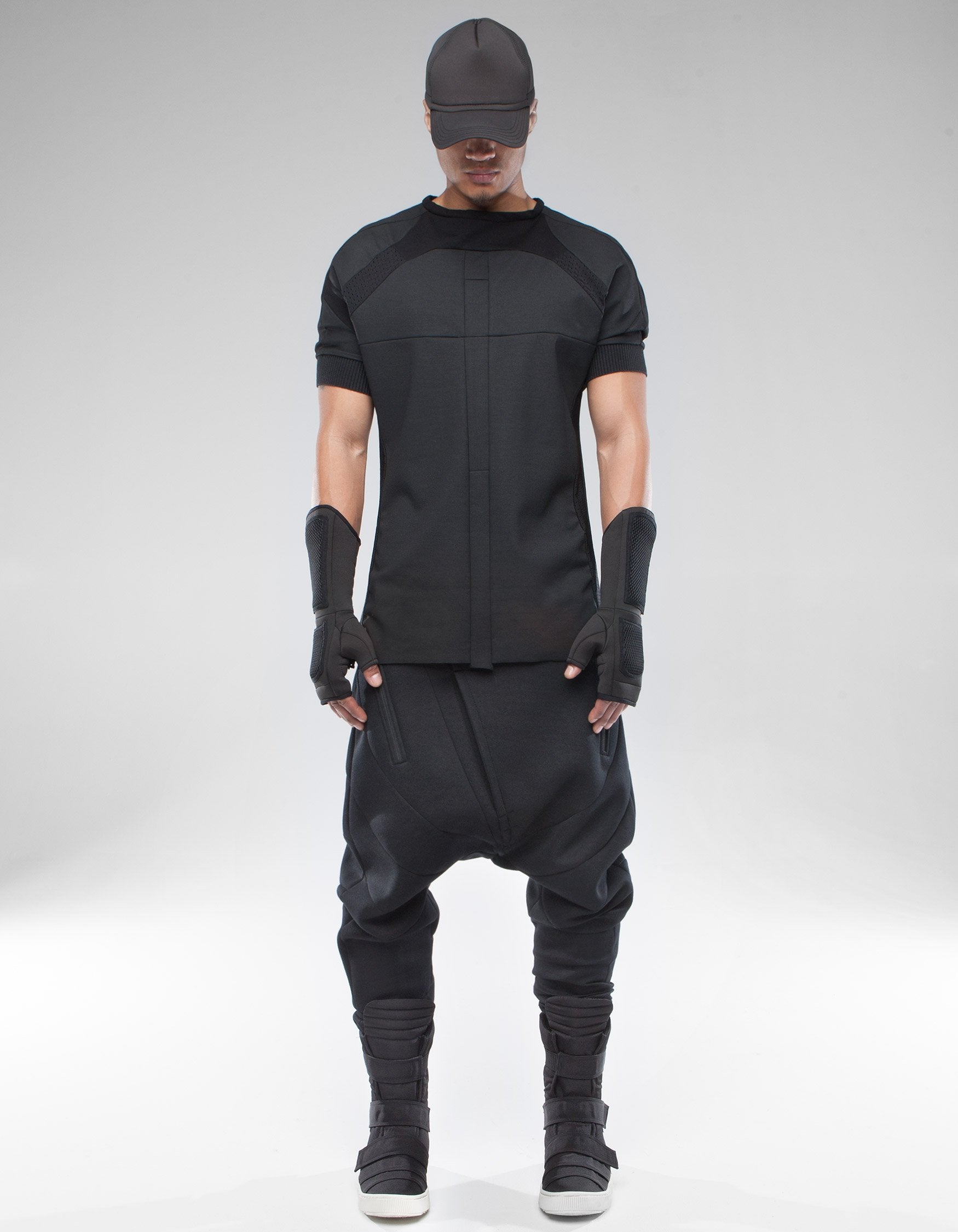In this image, a man stands against a light gray background, modeling an all-black outfit with distinct, intricate details. He is centered in the frame and is looking downwards, obscuring his eyes with a black baseball cap. His attire includes a short-sleeved black shirt featuring a unique vertical rectangle thread design down the center. His arms are adorned with extended black gloves resembling MMA gloves that reach his forearms, enhancing his muscular build. His black pants are baggy, reminiscent of ninja-inspired clothing, contributing to an overall Asian-inspired aesthetic. The outfit is complemented by tall black boots with white soles and straps wrapping around them, adding a striking contrast to the monochromatic ensemble.